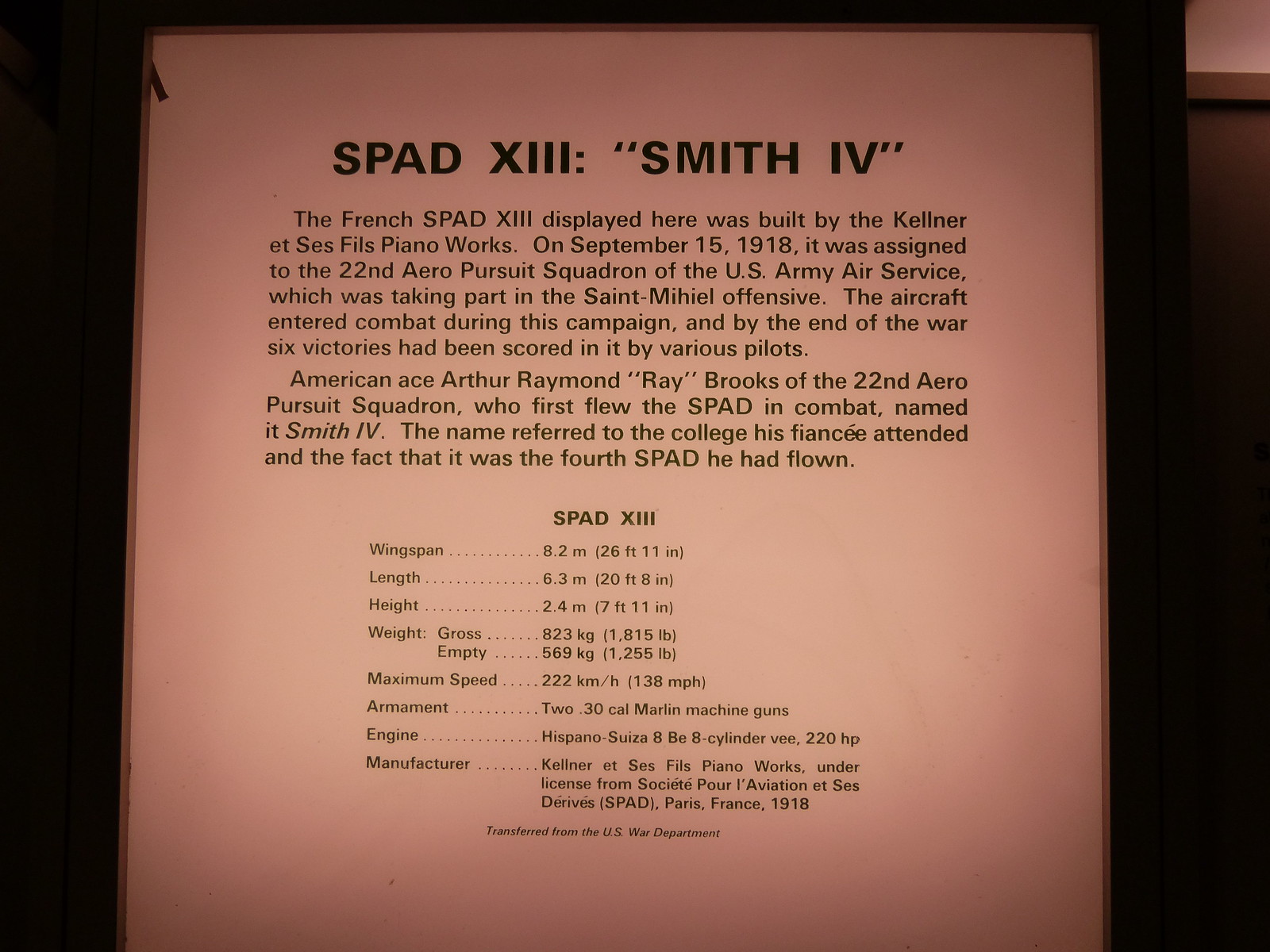This is a photograph of a framed plaque, slightly discolored to a pinkish-peach hue due to age, detailing the French SPAD XIII, also labeled as "Smith IV" in Roman numerals. The SPAD XIII, built by the Kellner-Éts & Filz Piano Works on September 15, 1918, was assigned to the 22nd Aero Pursuit Squadron of the U.S. Army Air Service. This squadron was actively engaged in the St. Mihiel Offensive during World War I. Notably, American ace Arthur Raymond "Ray" Brooks piloted this aircraft, naming it "Smith IV" in honor of his fiancée's college and as a marker of it being the fourth SPAD he had flown. By the end of the war, the plane had achieved six victories. The plaque not only narrates this history but also includes technical specifications such as wingspan, length, height, weight, maximum speed, armament, engine, and manufacturer details.